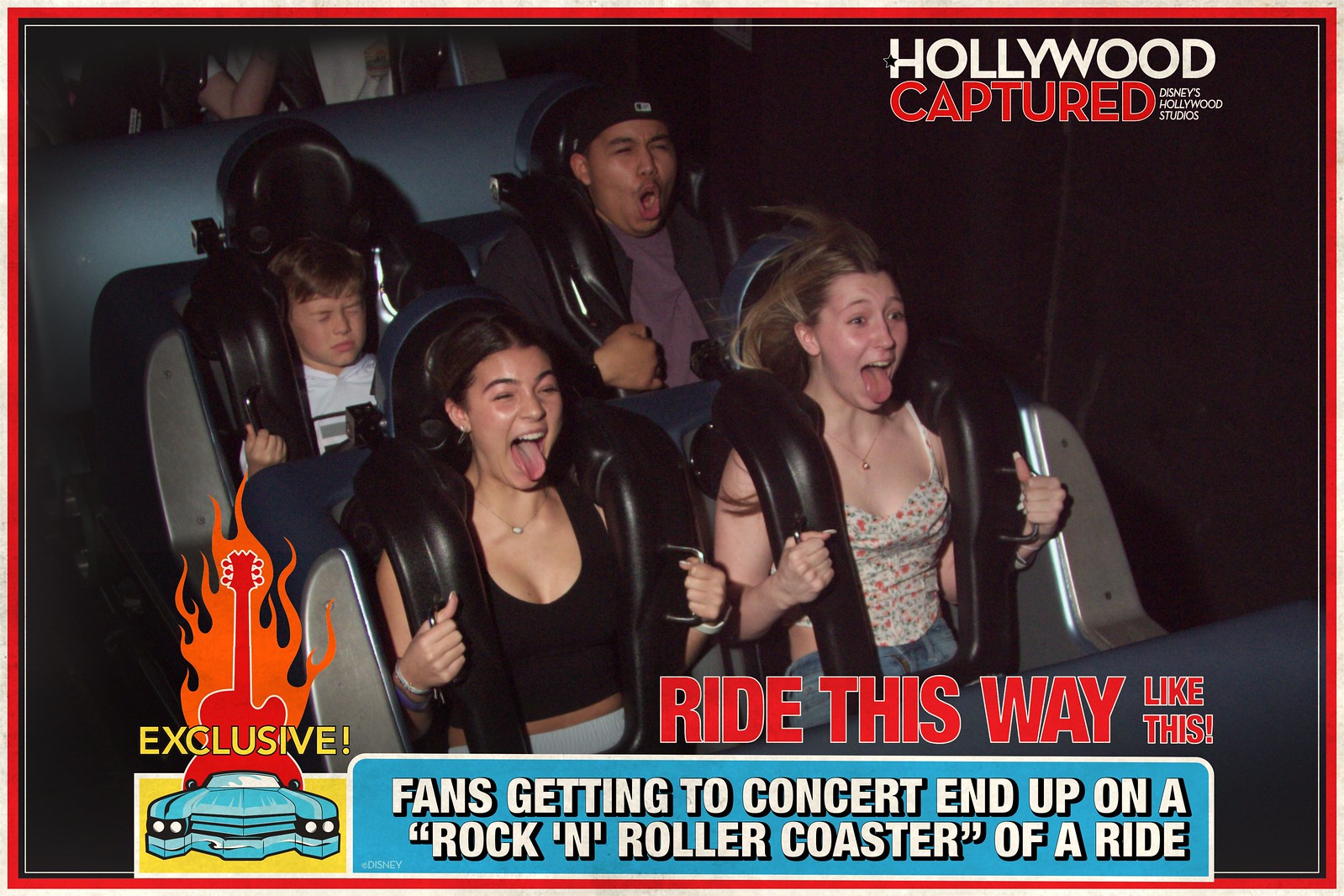The photograph captures four individuals experiencing the thrill of an amusement park ride, likely a rollercoaster. Seated in two rows of two, the front row features two teenage girls with their mouths wide open and tongues playfully sticking out, their hair wildly flying in the wind. In the back, a young child on the left is keeping his eyes tightly shut, while a man on the right, wearing a hat, appears to be howling with excitement, his mouth forming a large "O". The image, seemingly taken during a nighttime ride, includes a text overlay at the top right that says "Hollywood Captured" and "Disney's Hollywood Studios." At the bottom, there is a caption in red letters, "ride this way like this," followed by white text on a blue background that reads, "fans getting to concert end up on a rock and roller coaster of a ride." The photo is framed with a red border, and in the lower-left corner, there’s a vibrant cartoon image of a red guitar with orange flames, labeled "exclusive" in yellow letters, alongside a cartoon drawing of the front end of a big car.